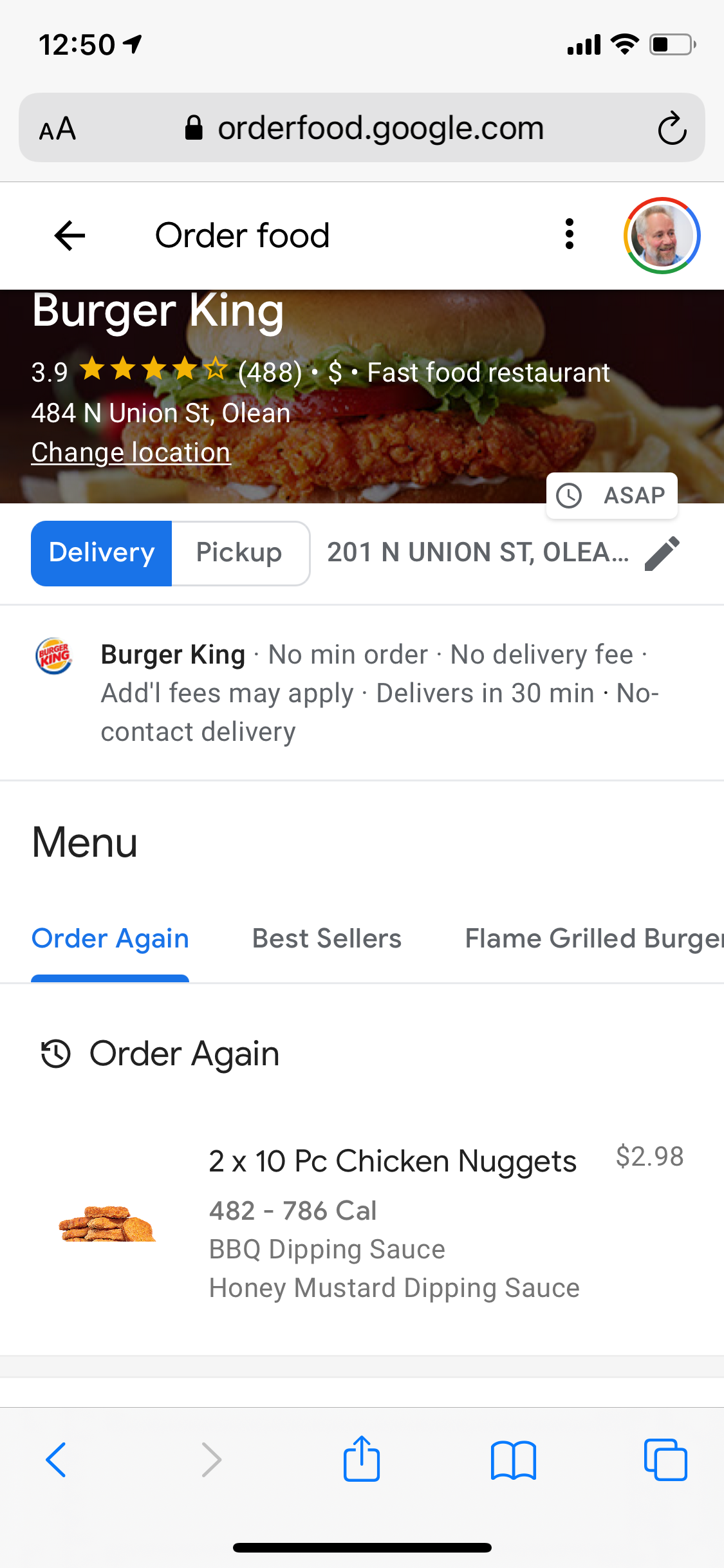An elderly man with gray hair and a beard is browsing the orderfood.google.com website on his smartphone. He is logged into his account, as indicated by his profile picture in the upper right corner of the screen. The restaurant currently displayed is Burger King, located at 484 North Union Street in Olean. The screen shows the "Order Again" tab highlighted in blue, indicating his previous order of two 10-piece chicken nuggets accompanied by barbecue and honey mustard dipping sauces. The top of the page prominently displays the Burger King name and features a mouth-watering image of a chicken sandwich garnished with tomato, lettuce, and what appears to be mayonnaise, surrounded by a heap of golden fries. The time displayed on the phone is 12:50, and the delivery option is highlighted in blue, suggesting that he might be considering placing another order soon.